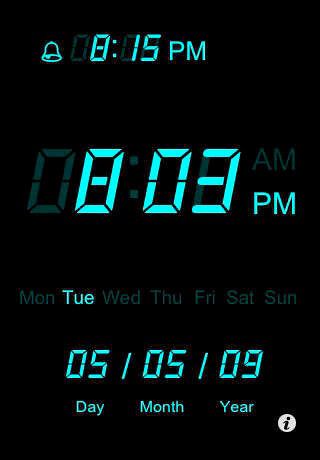The image displays a digital clock set against a black background, featuring a glowing turquoise or aqua-colored interface. In the upper left corner, there is a small bell symbol, followed by the time 8:15 p.m. Centrally located, the time is prominently displayed as 8:03 p.m. Below the central time display, the days of the week are listed in abbreviated form: MON, TUE, WED, THU, FRI, SAT, and SUN. The day "TUE" is illuminated, indicating it is Tuesday. Directly beneath this section, the date is displayed as 05-05-2009, denoting May 5th, 2009. The labels "day," "month," and "year" are inscribed beneath the date for clarity. In the lower right corner, there is a small information icon.